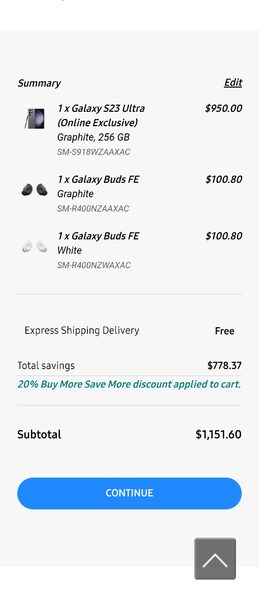Detailed Caption:

The image showcases a detailed summary of a purchase displayed within a sleek gray box, featuring items bought by a customer. The box has a "Summary" label positioned at the top left corner and an "Edit" option on the top right corner. Here's an itemized breakdown of the purchases:

1. **Galaxy S23 Ultra**: This flagship phone, available exclusively online in a stunning graphite color, comes with 256GB of storage and costs $950.
2. **Galaxy Buds FE (Graphite)**: A pair of wireless earbuds in a matching graphite hue, priced at $100.
3. **Galaxy Buds FE (White)**: Another pair of wireless earbuds but in a crisp white color, individually priced at $100.80.

The summary also notes that express shipping for the order is free, and the total savings amount due to discounts is a substantial $778.37. Notably highlighted in green, a 20% "Buy More, Save More" discount has been applied to the cart, enhancing the overall value. The subtotal, after discounts, amounts to $1,151.60.

Below the itemized list, there is a prominent blue button labeled "Continue" for proceeding with the purchase. At the very bottom of the box, a gray square with a white upward-pointing arrow is visible, although its function is not specified. This comprehensive summary highlights a significant purchase involving high-tech devices and a notable discount, complete with free delivery.